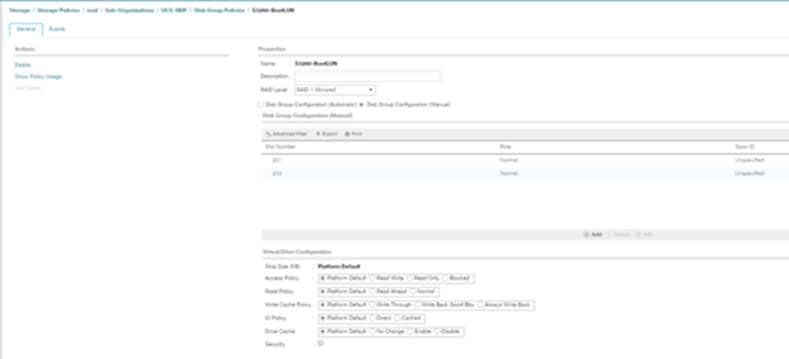The image displays a webpage, presumably related to the "Rayon" platform, featuring a somewhat complex layout. The top left corner showcases a series of listed locations labeled from 1 to 7. The area beneath this includes several tabs with illegible, blurry text, hinting at further navigational options. Adjacent to these tabs, more text appears, again blurry and blue, with only the word "properties?" discernible. Within this section, there is a reference to "name," "description," "read layer," and other pieces of indistinct text, suggesting this page might pertain to certain configurable settings.

To the right of this is a comprehensive table, presenting what looks like rows of data. At the bottom right of this table, there are visible rows, numbered similarly from 1 to 7. Each row seems to have various attributes: the first row has 4 attributes, followed by 3 attributes, then another with 4 attributes, and so on. The last row appears to end with an attribute labeled "security," accompanied by a positive checkmark. However, due to the blurriness, the exact context remains challenging to ascertain.